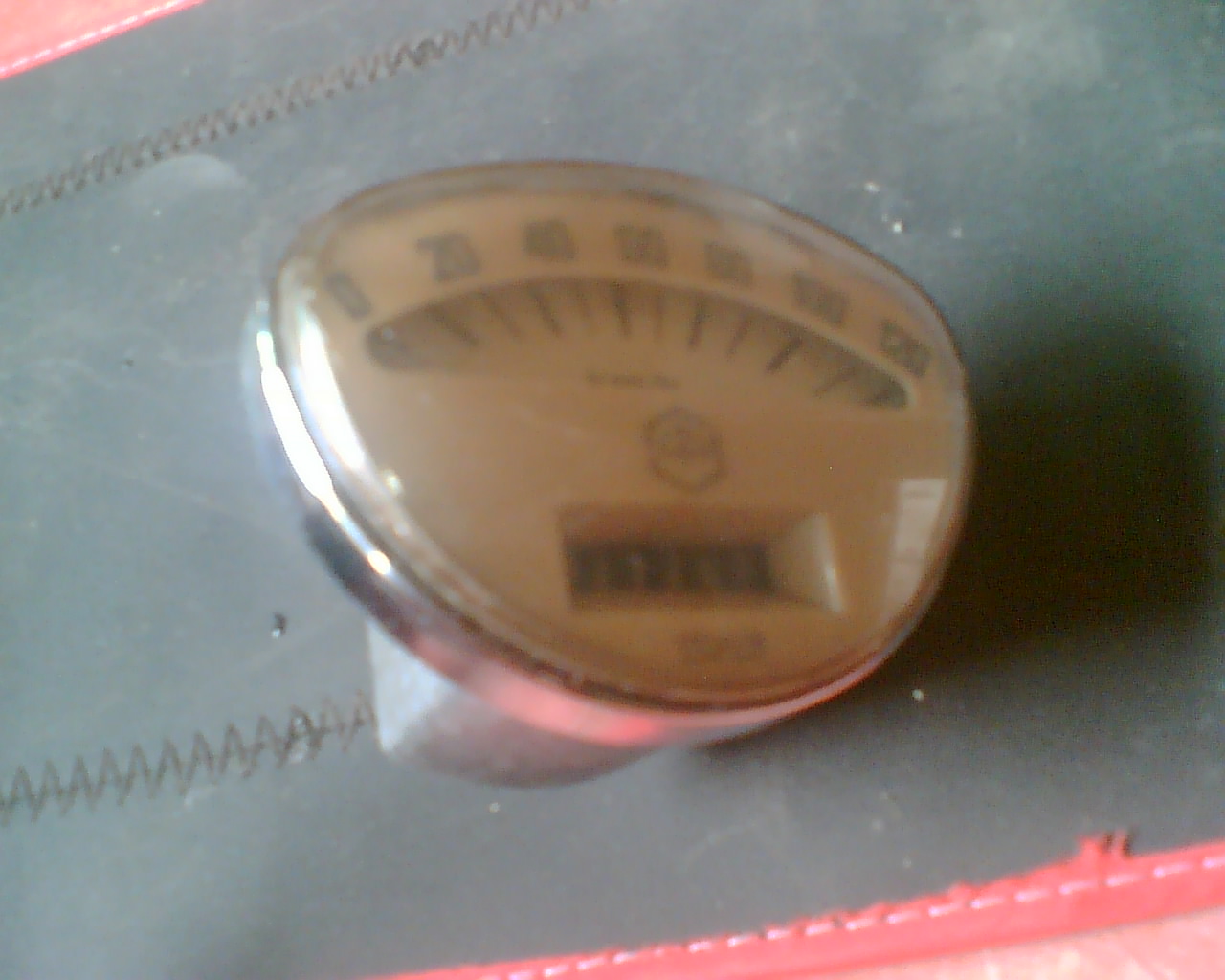The image appears to be an old, possibly analog photograph showcasing a teal leather or fabric background with a prominent zigzag stitch pattern. The top and bottom edges feature a coral-colored fabric trim with straight stitching. At the center of the photo is an indistinct device that resembles an odometer or counting mechanism. This device has a silver housing and a transparent plastic cover over a beige dial marked with the numbers 0, 20, 40, 60, 80, 100, and 120. There is a gauge needle, likely used to indicate measurements or counts, and a hexagonal icon. Below the dial, there is a section akin to an odometer, with unreadable black rolling indicators, possibly signifying distance or counts. Beneath this section, there is also some illegible text. The exact purpose of the device remains unclear, with potential uses ranging from sewing to general counting or pacing functions.